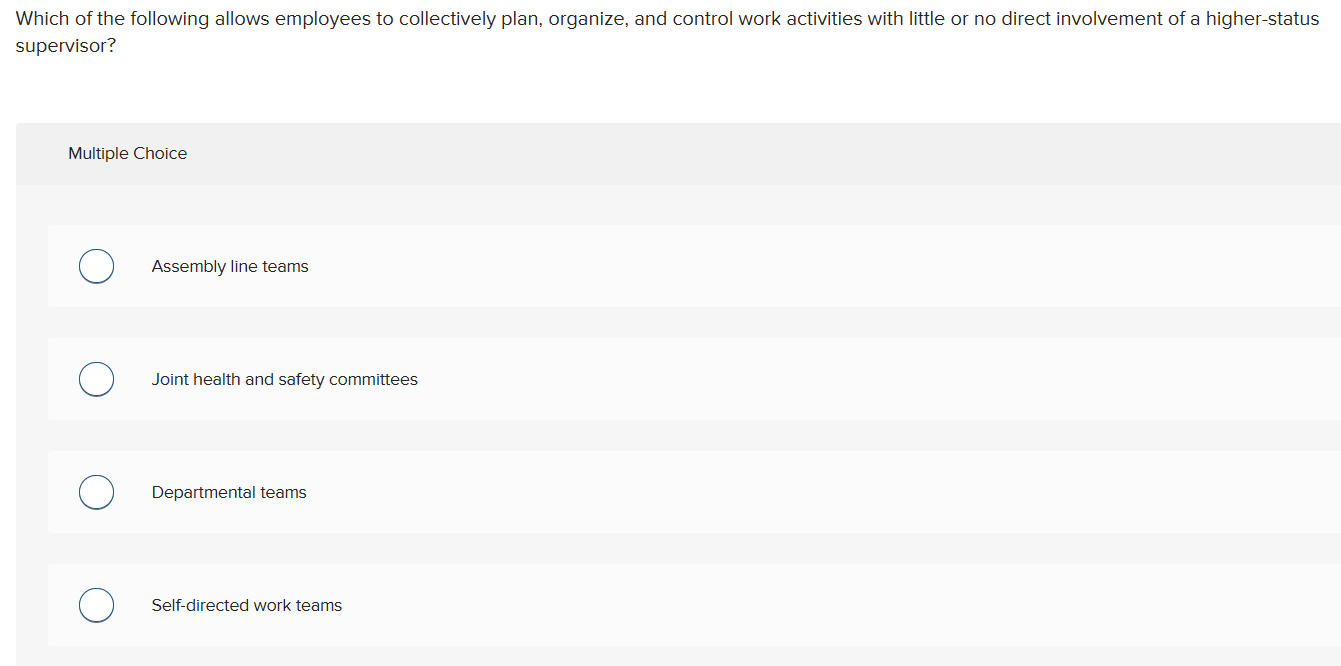The image depicts a multiple-choice interface on a gray background. The top section features a darker gray header with the text "Multiple Choice" located in the top left corner. Below this header, the rest of the screen is a lighter gray.

At the very top, there is a question in a white section, which reads, "Which of the following allows employees to collectively plan, organize, and control work activities with little or no direct involvement of high-status supervisors?"

Underneath the question, there are four options presented in a vertically layered format. Each option is represented by a white clickable bubble, followed by the respective text in black:

1. "Assembly line teams"
2. "Joint health and safety committees"
3. "Department teams"
4. "Self-directed work teams"

Users can select any of these four options, indicating their choice by clicking on one of the white circles next to the text.